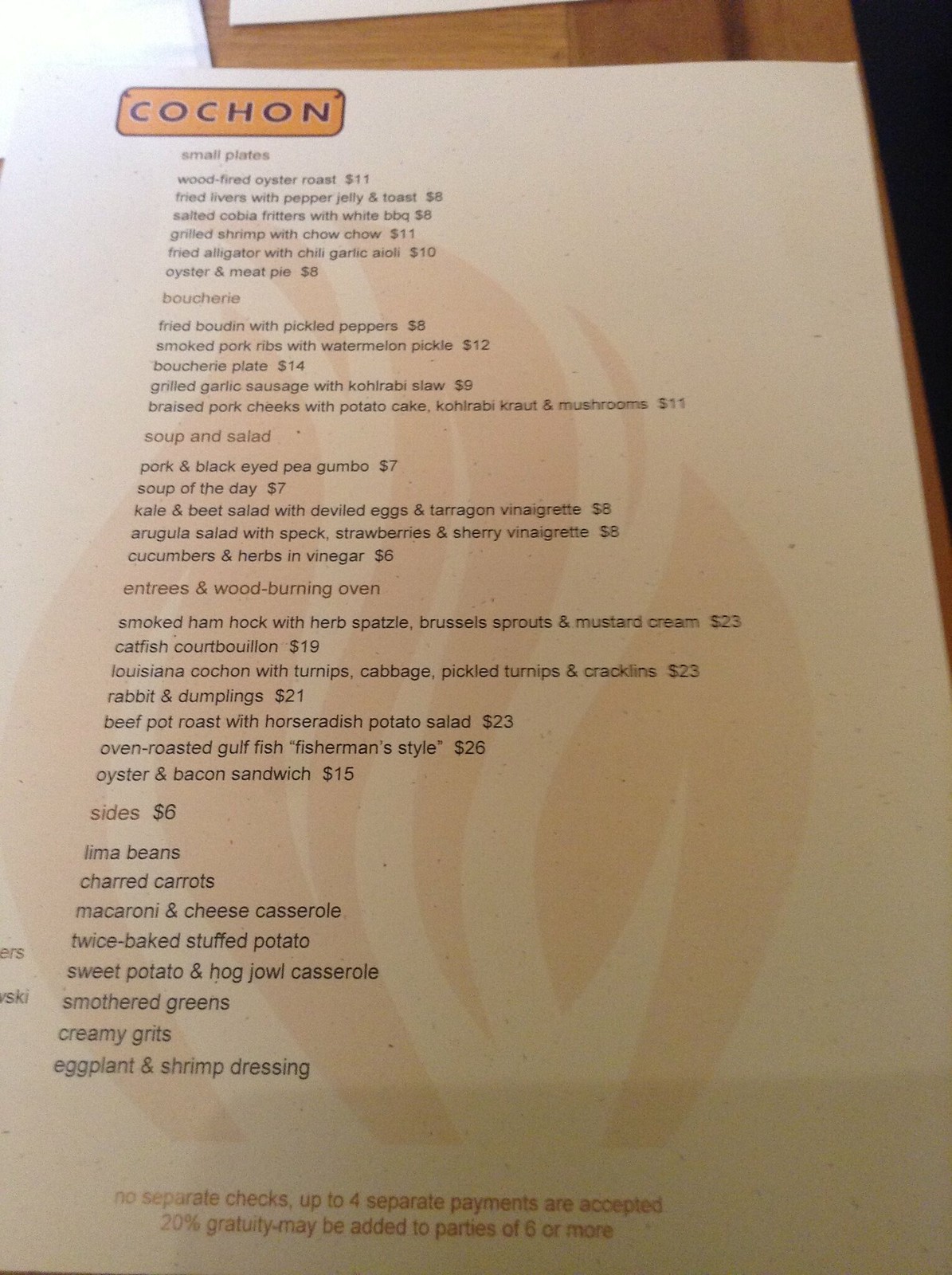This is a detailed description of a white menu page for a restaurant named Cochon. The top left corner of the menu features the logo, which consists of an orange rectangle with rounded corners, containing the letters "COCHON" in all capital letters and dark brown lettering.

The menu is divided into several sections, starting with "Small Plates":
- Wood-Fired Oyster Roast: $11
- Fried Livers with Pepper Jelly and Toast: $8
- Grilled Shrimp with Chow Chow: $11
- Fried Alligator with Chili Garlic Aioli: $10
- Oyster and Meat Pie: $8

Next is the "Butchery" section:
- Fried Boudin with Pickled Peppers: $8
- Smoked Pork Ribs with Watermelon Pickle: $12
- Butchery Plate: $14
- Grilled Garlic Sausage with Kohlrabi Slaw: $9
- Braised Pork Cheeks with Potato Cake, Kohlrabi, Kraut, and Mushrooms: $11

Following that, the "Soup and Salad" options are:
- Pork and Black-Eyed Pea Gumbo: $7
- Soup of the Day: $7
- Kale and Beet Salad with Deviled Eggs and Tarragon Vinaigrette: $8
- Arugula Salad: $8
- Cucumbers and Herbs in Vinegar: $6

Under the section "Entrees and Wood-Burning Oven," the offerings include:
- Smoked Ham Hock: $23
- Catfish: $19
- Louisiana Cochon: $23
- Rabbit and Dumplings: $21
- Beef Pot Roast: $23
- Oven-Roasted Gulf Fish Fisherman Style: $26
- Oyster and Bacon Sandwich: $15

The "Sides" section lists a variety of accompaniments, each priced at $6:
- Lima Beans
- Charred Carrots
- Macaroni and Cheese Casserole
- Twice-Baked Stuffed Potato
- Sweet Potato and Hog Jowl Casserole
- Smothered Greens
- Creamy Grits
- Eggplant and Shrimp Dressing 

This detailed menu vividly portrays the diverse and appealing culinary offerings available at Cochon.